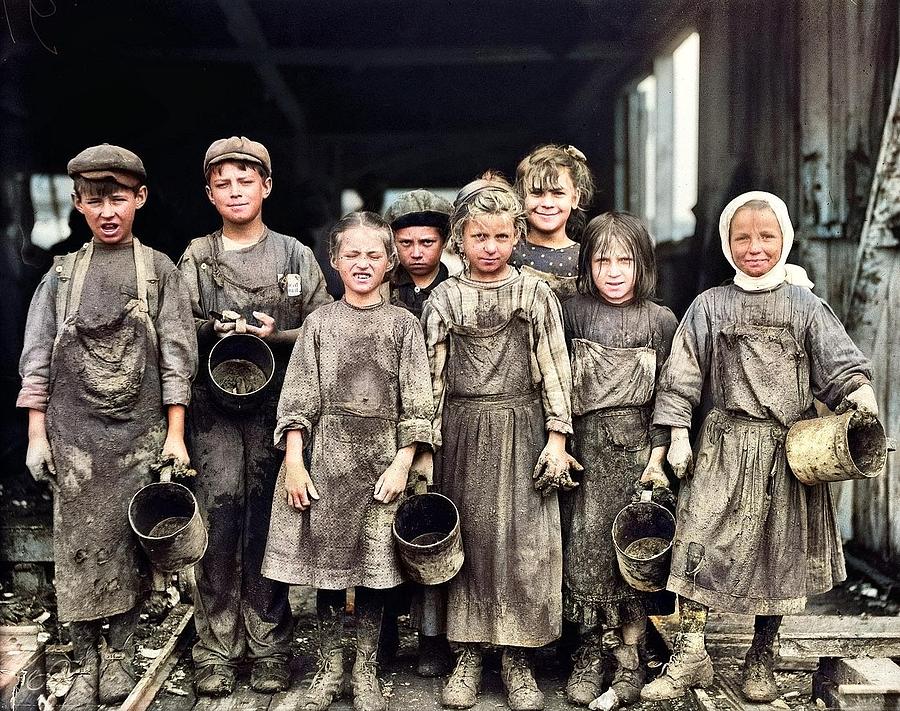This is a colorized vintage photograph, likely from the early 20th or late 19th century, depicting eight young child laborers, around 11 years old or younger, standing at the entrance of a dirty, dimly lit building. The children are a mixture of boys and girls, with some wearing caps and one girl having her head and neck wrapped in a white scarf. They are all dressed in soiled clothing and aprons, covered head-to-toe in mud, and are holding metal buckets with muddy contents. The ground beneath them appears to be a railway, suggesting an industrial setting. Most of the children are smiling despite their grimy appearance, though one child at the back looks particularly unhappy. The background of the building gets progressively darker towards the rear, with some light filtering in through the windows at the back and sides.